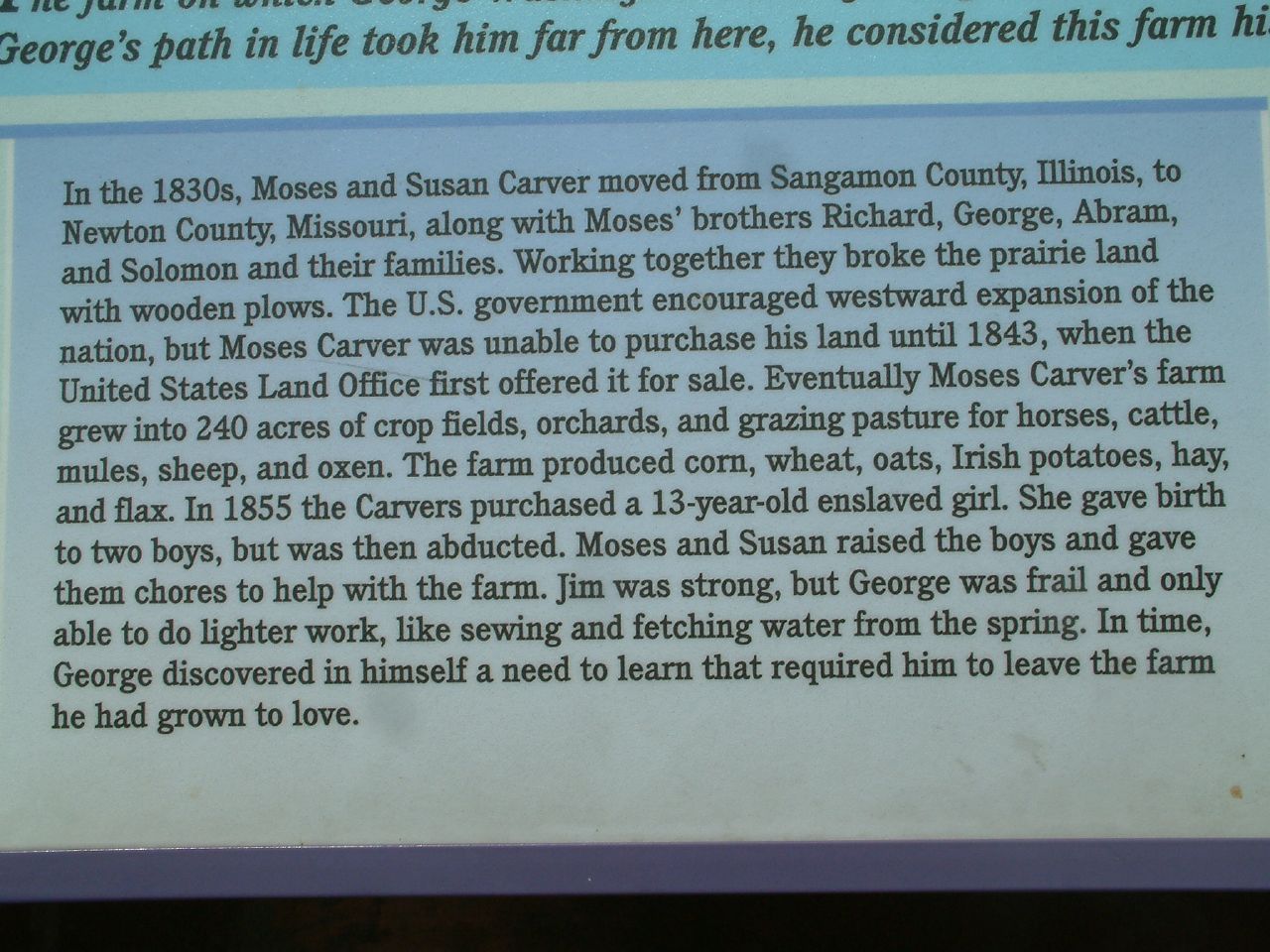This image captures a page from a book with light blue font. The excerpt provides a historical account, starting with Moses and Susan Carver who moved from Sangamon County, Illinois to Newton County, Missouri in the 1830s. They were accompanied by Moses' brothers Richard, George, Abram, and Solomon and their families. Together, they broke the prairie land with wooden plows, spurred by the U.S. government's encouragement of westward expansion. However, Moses Carver couldn't purchase his land until 1843, when the United States Land Office first offered it for sale. Over time, Moses Carver's farm expanded to 240 acres including crop fields, orchards, and grazing pastures for horses, cattle, mules, sheep, and oxen. The farm yielded corn, wheat, oats, Irish potatoes, hay, and flax.

In 1855, the Carvers purchased a 13-year-old enslaved girl who later gave birth to two boys before being abducted. Moses and Susan took in these boys, assigning them chores on the farm. Jim proved strong and capable of hard labor, while George, being frail, was limited to lighter tasks like sewing and fetching water. Eventually, George's yearning for education led him to leave the farm, a place he had cherished and grown to love.